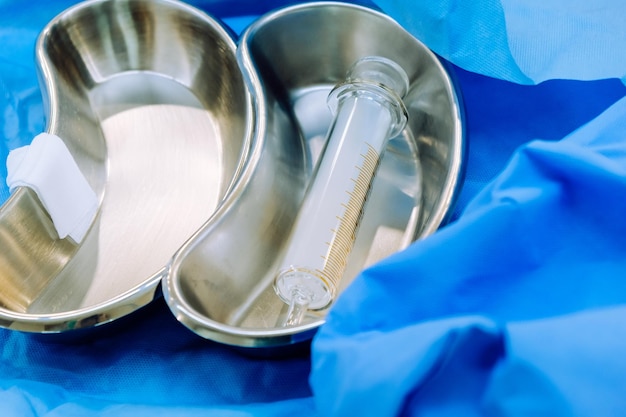This is a detailed and sharp indoor photograph taken from above, depicting a medical setup. Centered in the image, resting on a bright blue medical cloth that is slightly bunched and transitions from dark to light blue, are two kidney-shaped, stainless steel dishes positioned towards the left-hand side. The dish on the left has a small rectangular piece of gauze or a possibly wet cloth draped over its inner curved edge. The dish on the right contains a clear, glass syringe with nothing inside it; the plunger is fully depressed, and it appears brand new, with gradient markings in orange. Some confusion exists over whether the syringe contains an opaque white substance, however this is not universally agreed upon in the interpretations. The silver metallic dishes and the vibrant blue cloth create a sharp and clear contrast, with no text or other elements visible in the background, highlighting the medical equipment in the photograph. The blue cloth evokes the attire and fabric commonly seen in hospital settings, enhancing the medical tableau.